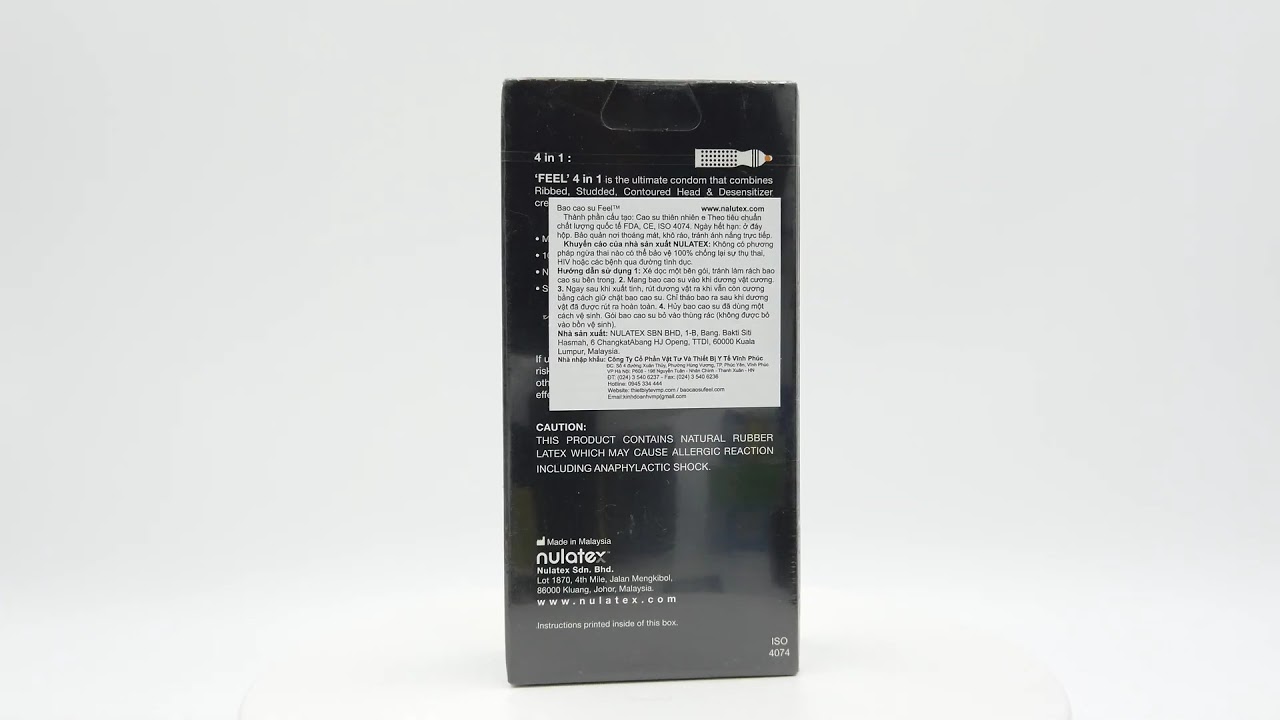The image depicts a rectangular product label featuring a prominent black box at its center, filled with multiple lines of white text. This black box occupies about a third of the label's height and stands against a grayish-white background. The text within the black box includes critical cautionary statements, noting that the product contains a natural flavor that could cause allergic reactions, including anaphylactic shock. Additionally, there are specific identifiers such as "Nulatex," "4-074" located towards the bottom, and "4N1" positioned at the top. Beside this information, there is a small white square with black text that is difficult to decipher due to its size and blurriness. In the upper right-hand corner, the image features an object resembling a white magic marker or tool with its cap off. Additional details include the product being manufactured in Malaysia, with the words "no late" noted near the lower left-hand corner, alongside an address and web address. Overall, the label provides detailed product information, ingredients, usage instructions, and manufacturer's details.